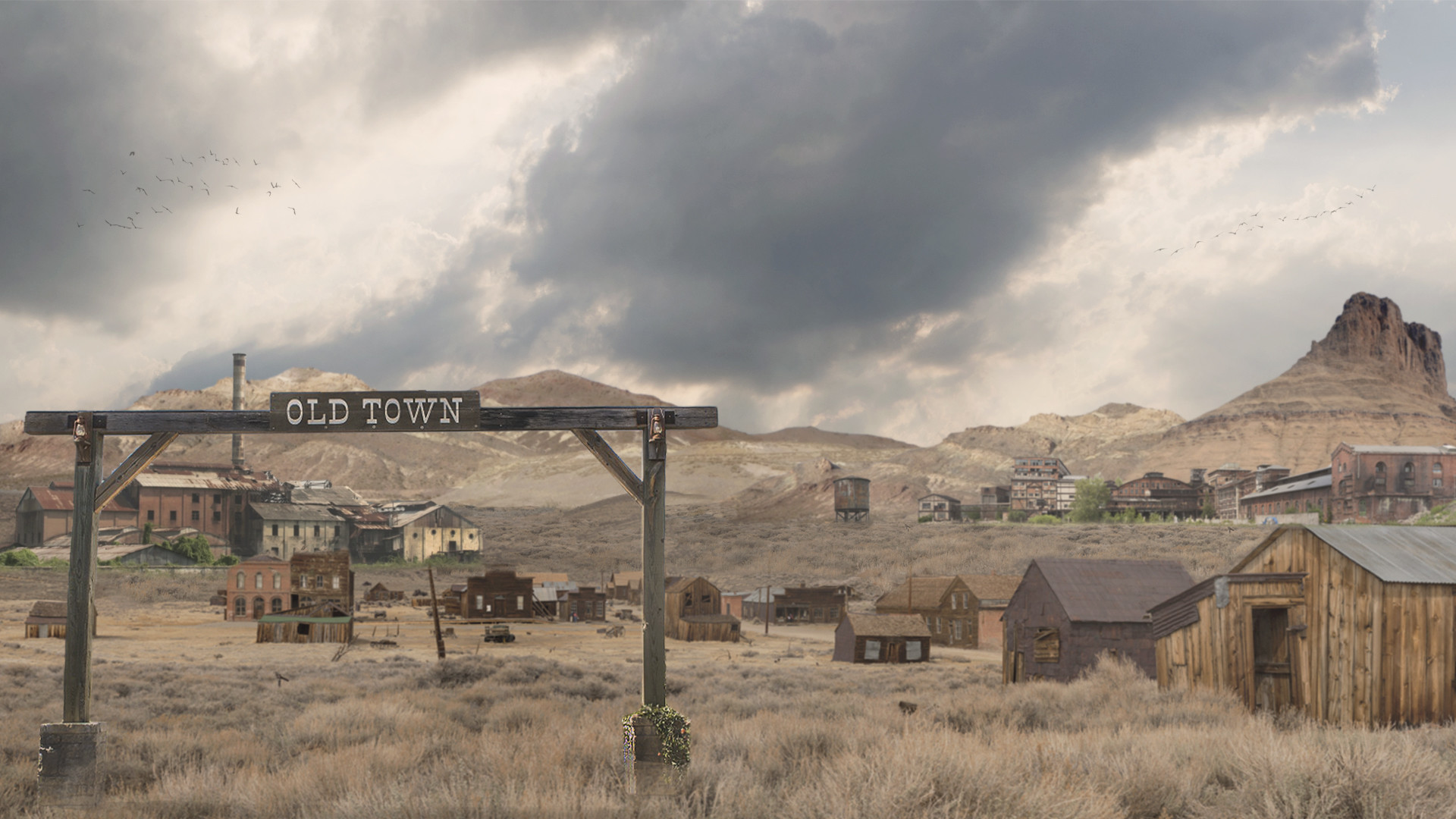This evocative photograph, reminiscent of the old days, captures a somber, cloudy scene of an old western ranch town. Dominating the foreground is a prominent sign arching over the entrance, reading "Old Town," set against a backdrop of dry, high grass. The town consists of a series of rustic, wooden buildings, ranging in color from brown to brick red and a few in white. These humble structures, which include barns and houses, evoke the atmosphere of a movie set. In the distance, a rocky mountain range looms beneath a dark, cloud-laden sky, creating a sense of impending rain. A flock of birds dots the gloomy sky, contributing to the desolate ambiance. The terrain transitions from the flat, grassy expanse at the front to the hilly and rugged landscape beyond, with no people visible in this haunting, timeless scene.